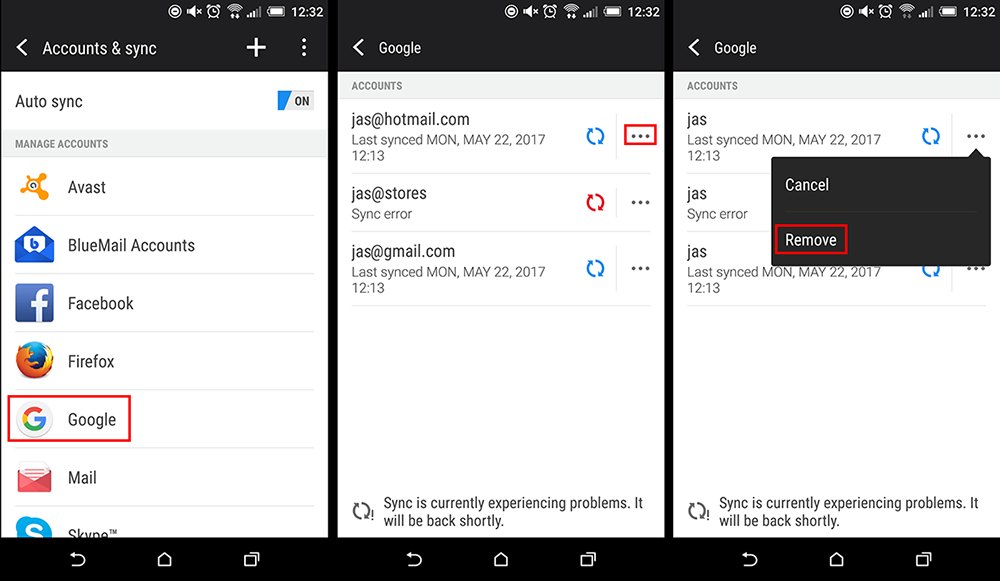**Descriptive Caption:**

The image comprises three screenshots from a mobile device, each displaying detailed information about account sync settings and statuses. 

**Left Screenshot:**
- **Top Bar:** Features a series of icons starting from left to right: a circular icon, a muted volume symbol, an alarm clock, a Wi-Fi signal, cellular signal (three out of five bars), a battery icon, and the time "12:32".
- **Main Content:** Displays the "Accounts and Sync" settings screen. At the top, there is a back arrow, a plus icon, and three vertical dots. Below, it states "Auto-sync is on".
- **Options:** Includes "Manage Accounts" followed by a list of accounts, each with its corresponding logo:
  1. Avast (with Avast logo) 
  2. BlueMail (with BlueMail logo)
  3. Facebook (with Facebook logo)
  4. Firefox (with Firefox logo)
  5. Google (with Google logo)
  6. Mail (with Mail logo)
  7. Skype (with Skype logo)

**Center Screenshot:**
- **Top Bar:** Identical to the left screenshot.
- **Main Content:** Shows the "Google" account sync settings screen. At the top, a back arrow is present.
  - First Account: "jazz at hotmail.com", last synced on Monday, May 22, 2017, at 12:13.
  - Second Account: "jazz at stores", with a sync error message.
  - Third Account: "jazz at gmail.com", last synced on Monday, May 22, 2017, at 12:13. Below, it states, "Sync is currently experiencing problems. It will be back shortly."

**Right Screenshot:**
- **Top Bar:** Again, identical to the previous screenshots.
- **Main Content:** Repeats the Google account screen from the center screenshot, but with the three vertical dots (menu) pressed, opening a dropdown menu. 
  - The dropdown menu shows two options in a black text box: "Cancel" and "Remove", with "Remove" being highlighted in a red square. 

**Overall Context:** These images collectively show the navigation and status of account synchronization settings on a mobile device, focusing on various accounts and detailed sync status for Google accounts.